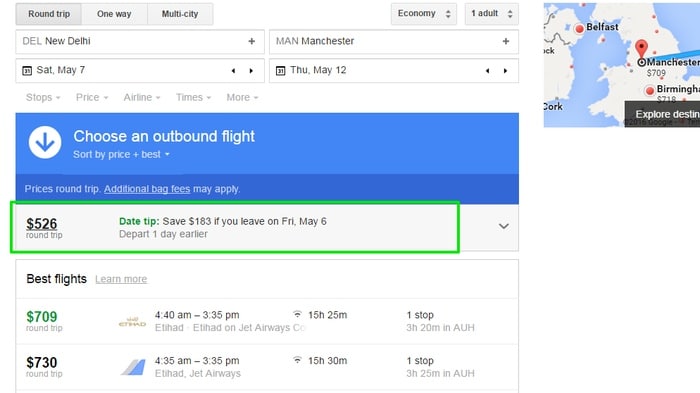This image showcases a detailed layout of a flight booking page. At the top left, there are three tabs labeled "Round trip," "One way," and "Multi-city." On the top right, two additional tabs read "Economy" and "1 adult." Below these, the origin and destination are displayed: "New Delhi" on the left and "Manchester" on the right, with the travel dates specified underneath as "Saturday, May 7th, to Thursday, May 12th."

A gray section below this offers five filter categories: "Stops," "Price," "Airline," "Times," and "More," listed from left to right. Underneath this filter bar is a prominent blue section featuring the text "Choose an outbound flight," accompanied by a white circle and a blue arrow pointing downwards to the left.

Further down, a dark blue banner states, "Prices are round trip, additional bag fees may apply." Beneath this in a green background, the price "$526" is highlighted, along with a note indicating a potential savings, "Save $183 if you leave on Friday, May 6th. Depart one day earlier."

The section labeled "Best flights" presents times and durations for the two highlighted options. The first flight is scheduled from 4:40 AM to 3:35 AM, and the second from 4:35 AM to 3:35 PM, lasting 15 hours and 25 minutes and 15 hours and 30 minutes respectively. Both flights are marked with "One stop" in a white background.

The comprehensive details conclude the image description.